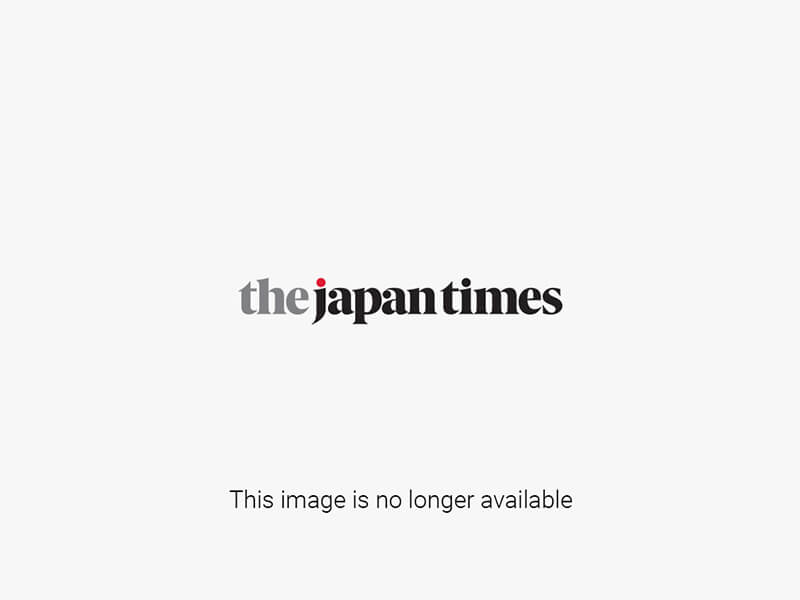The image captures a bustling scene of tourists gathered in front of an intricately carved snow or ice sculpture resembling a grand castle or mansion. This impressive structure, reminiscent of landmarks like Buckingham Palace, stands about 15-20 feet tall and stretches approximately 40 feet in length. The sculpture is adorned with detailed features such as roofs and sculpted pieces, and it emits a distinct wintry charm. In the foreground, a young Asian couple is seen taking a selfie, while numerous other visitors, many of whom are wearing masks and winter jackets, również are capturing memories of the event. The background reveals a modern urban landscape with towering skyscrapers and leafless, snow-dusted trees set against a bright blue sky with scattered clouds. Additionally, two flags are notable near the sculpture, one being the British flag and the other the Japanese flag, indicating an event of some significance. The scene is lively and well-lit, contributing to the overall clarity and visibility of the image.